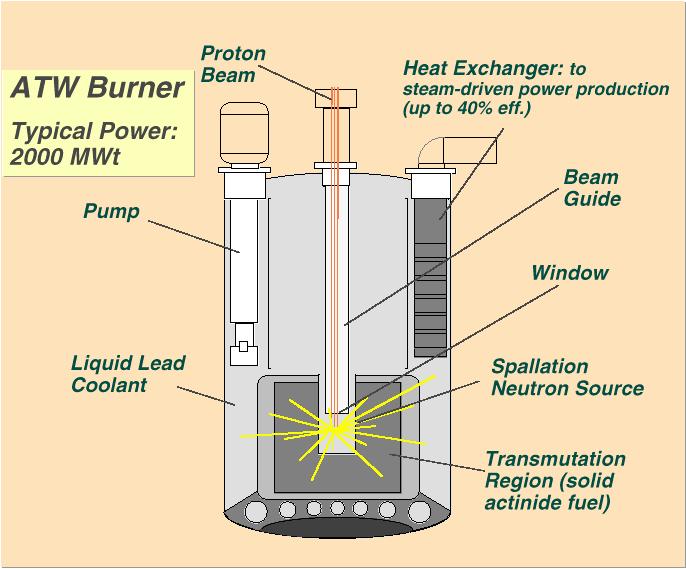This detailed diagram illustrates a typical ATW (Accelerator-Driven Transmutation of Waste) burner unit with a power capacity of 2000 MWT, presumably megawatts. The diagram, set against a peach-colored background, is dominated by a central cylindrical machine resembling a can, which is identified as the ATW burner. The detailed component labels are in italicized text, with each key part connected by lines from the burner to the label.

On the left side of the burner, labels identify the pump and the liquid lead coolant, whereas the top section highlights the proton beam, with the beam guide located near the center. Also prominently featured is a window at the front of the burner. The right side of the cylinder lists several other critical components: a heat exchanger for steam-driven power production with up to 40% efficiency, a spallation neutron source, and, at the bottom, the transmutation region containing solid actinide fuel. Sparks emanating from the bottom center of the cylinder suggest an active reaction occurring within the unit.